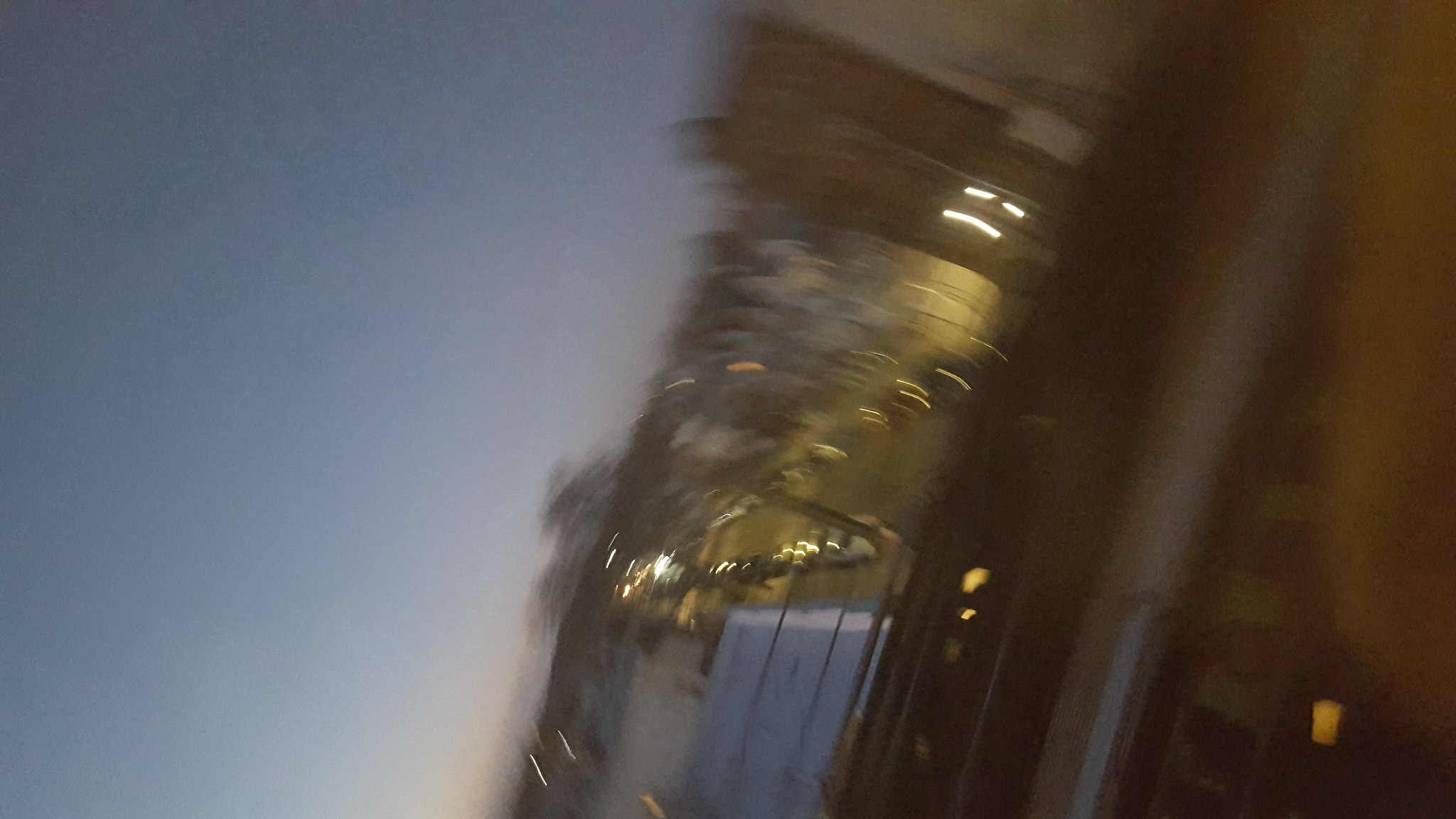A blurry, rectangular photograph captures a cityscape at dusk from an inclined angle. The top and bottom sides of the image are longer than the left and right sides. The left half of the image showcases a dark blue sky blending into an orange hue near the horizon, indicating either dusk or the onset of night. The right half presents an aerial view of a city street as seen from a balcony. Dominated by a dark metal railing at the forefront, the city street below features light gray asphalt free of any markings, with several cars parallel parked on both sides. The street is flanked by multiple buildings on either side, illuminated by an array of streetlights casting yellow and white glows.